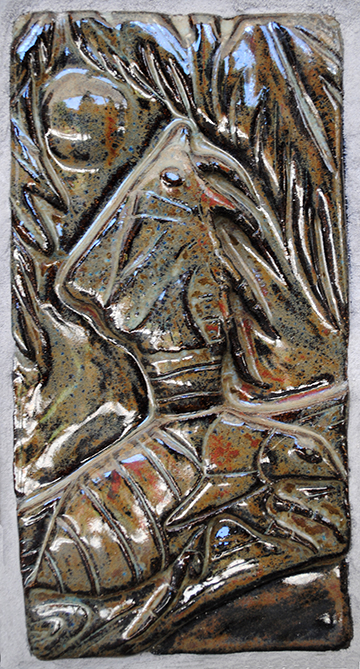The image depicts a tall, rectangular sculpture or plaque with a shiny finish, potentially crafted from metal or highly polished ceramic. The overall color palette consists of grays and browns with touches of blue at the top, and hints of reddish-orange and black. The artwork is abstract, featuring a central shape with a wide base that narrows into a triangle, reminiscent of a man’s head adorned with a cone-shaped headdress or a plant pushing up from the ground, blending with sun and grass motifs. The piece is adorned with stripes, lines, curves, and dimples, and toward the bottom, there is a pattern that might evoke the body of a bee. The intricate details and reflective surface add layers of visual complexity to the abstract composition.